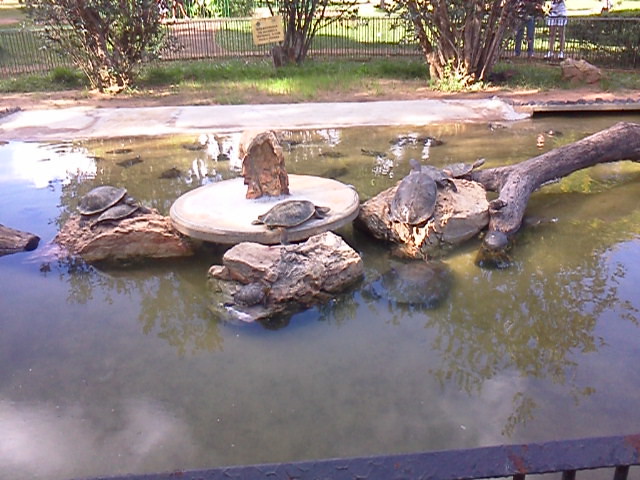The image captures an outdoor scene of a turtle enclosure, possibly in a reserve or zoo. Central to the enclosure is a round, concrete platform crowned with a large rock on which a turtle is basking. This platform is encircled by various large rocks, many of which serve as additional basking spots for the turtles. A prominent feature is a substantial tree branch that extends from the left side of the image, touching one of the rocks. 

The enclosure features a combination of green grass and water, the latter appearing somewhat murky with several turtles swimming within. Three trees are also visible inside the enclosure, contributing to the natural ambiance. 

In the background, a fence surrounds the entire area, and two people can be seen standing behind it in the top right corner. Additionally, a distant yellow or brown sign is mounted on a tree, though the details are indistinct due to distance and clarity. Natural sunlight illuminates the scene, highlighting the turtles and the general setting vividly.